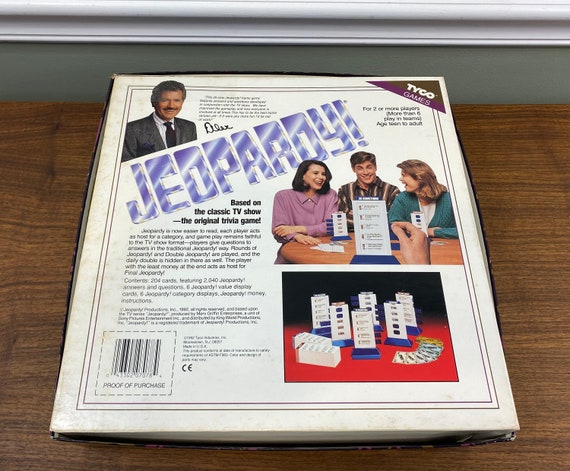The photograph captures the back of a slightly aged Jeopardy game box, laying on a dark brown wooden table with a gray-green wall featuring a white border at the top. The box, which has a white base with some yellowing and two thin black borders, is slightly angled with the bottom wider than the top. In the upper left-hand corner, there is an image of a smiling Alex Trebek, characterized by his grayish hair, mustache, gray suit jacket, and black tie. Adjacent to him, in the upper right-hand corner, a purple triangle with a brown bottom stripe displays the text "Tycho Games." Below Trebek's image, the word "Jeopardy" appears vertically slanted in vibrant electric purple letters with white streaks, giving it a shiny appearance.

Beneath the Jeopardy text, three individuals—two women and a man—are engrossed in playing the card game at a table, with the hand of a fourth person visible holding a game card displaying different clues. Lower on the box, another image depicts the cards and elements of the game setup. Text reading "based on the classic TV show, the original trivia game" is seen to the left of the players. In the bottom left-hand corner of the box, a barcode is labeled with "Proof of Purchase."